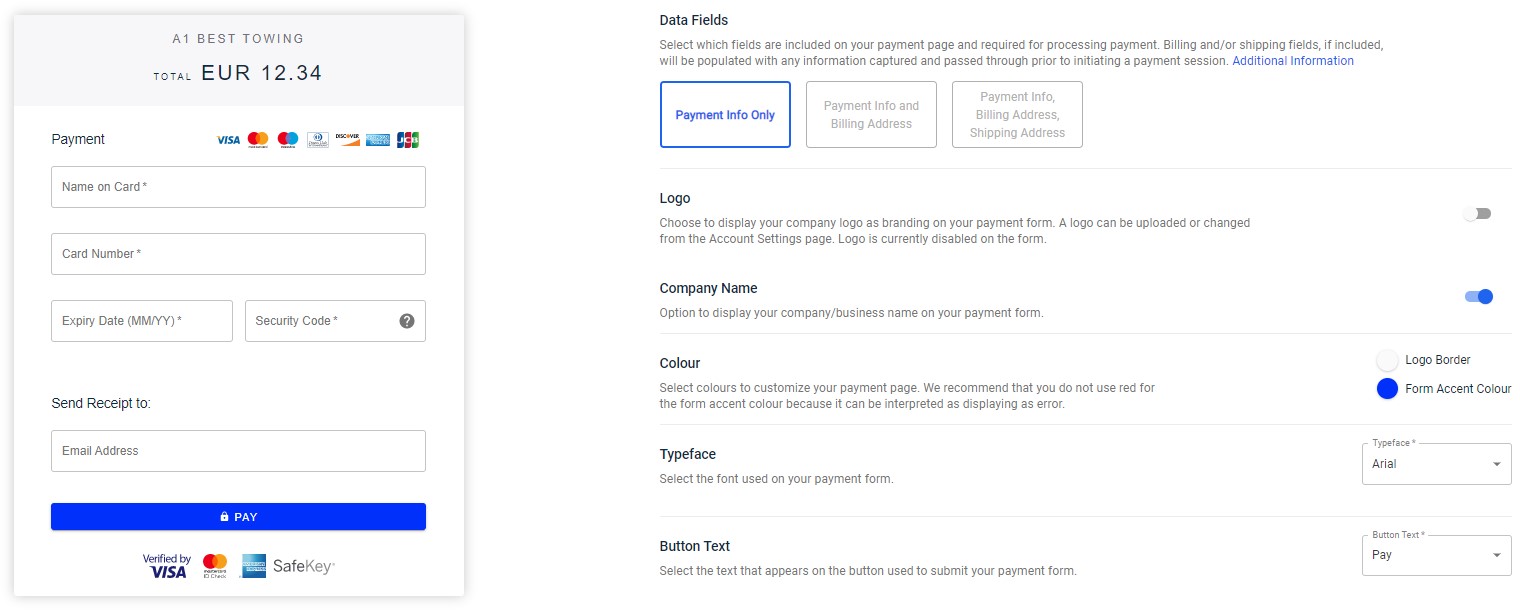This image showcases a split-screen screenshot, with the left panel displaying a payment form and the right panel showing design customization options for that payment interface.

The left panel, formatted in portrait orientation, features the payment form header labeled "A1 Best Towing" and the total amount due as €12.34. The form is designed to collect payments via major credit and debit cards. It includes fields prompting the user to input their name as it appears on the card, the card number, the expiration date, and the security code. Additionally, there is a field for entering an email address to which the receipt will be sent. The payment form is completed with a prominent blue button labeled "Pay" in white text at the bottom.

Meanwhile, the right panel is focused on the customization of the payment interface. It contains various data fields and options related to the design of the payment form. These customizable elements include the "Payment Info Only" highlighted box, followed by fields for the logo, company name, color, typeface, and button text, implying that this panel allows the user to tailor the payment interface to match their branding requirements. Overall, the image depicts the creator's process in designing a user-friendly and branded payment form for a towing service.